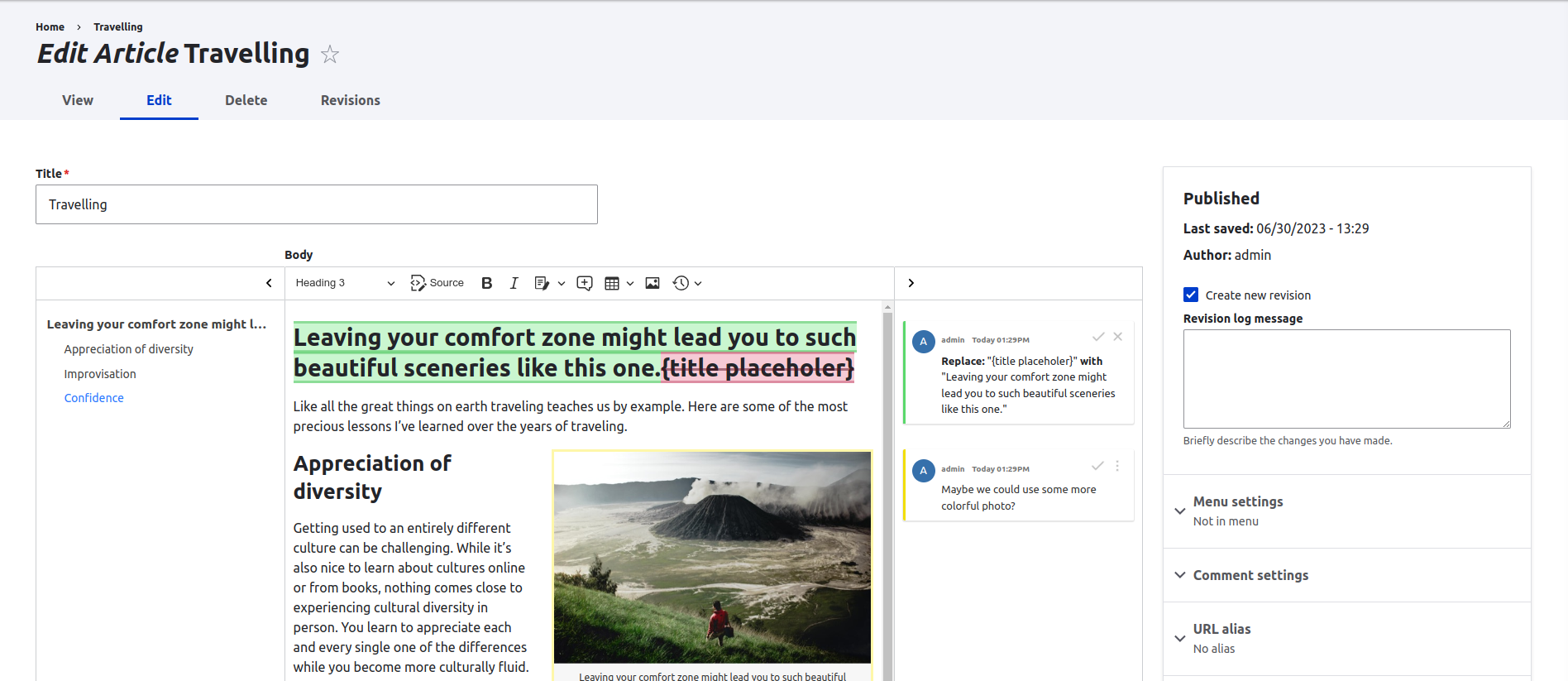**Detailed Caption:**

The image is a screenshot of a webpage featuring a white background throughout. In the top left corner of the page, "Home" is written in bold, followed by the word "Traveling" written underneath. Below this, prominently displayed, is "Edit Article: Traveling" in large, bolded text. Directly beneath are options labeled "View," "Edit," "Delete," and "Revisions," with "Edit" highlighted in blue, indicating it is the currently selected option.

Moving downwards, the text "Title" appears, accompanied by a red asterisk, implying that this section is required. In the title field, the word "Traveling" is entered. On the far left side of the page, the word "Published" stands out in large, black, bold letters, followed by the last saved date and time details. The "Author" is listed as "Admin."

In the central portion of the page, a section of a green-highlighted article is visible. The text within this green background is written in black and states, "Leaving your comfort zone might lead you to such beautiful sceneries like this one." Following this, text in red background with parentheses reads, "(title placeholder)." 

Below this, the article continues, with part of the text focusing on "Appreciation of Diversity," positioned to the left. To the right of this text, there is an image depicting a landscape that resembles a volcano.

This screenshot captures the editing view of an article about traveling, highlighting various sections of the webpage, partly in draft with placeholders, and visually indicating the user's interface for editing the content.